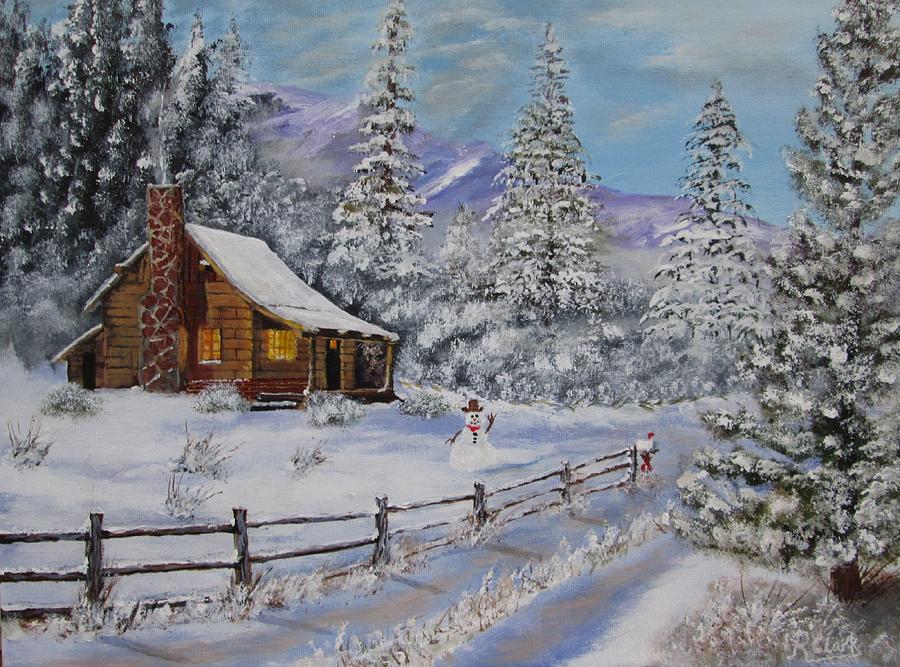This artwork depicts a serene winter scene featuring a log cabin made out of light brown natural wood, with a prominent red brick chimney bound by gray cement. Soft white smoke billows from the chimney, hinting at the warmth within, visible through the glowing lights inside the two windows and the front door's window. The cabin's roof and surrounding landscape are blanketed in snow, adding to the cozy ambiance. In the front yard stands a cheerful snowman adorned with a brown cowboy hat and a red scarf, one twig arm raised in greeting. Enclosing the yard is a wooden fence, also dusted with snow, which leads to a mailbox at its end. The scene is framed by large, snow-laden trees and further encircled by smaller plants within a snowy field. In the background, a light blue sky with white clouds lies above a range of purple mountains that peek from behind the tall pine trees, completing this picturesque and tranquil winter setting.